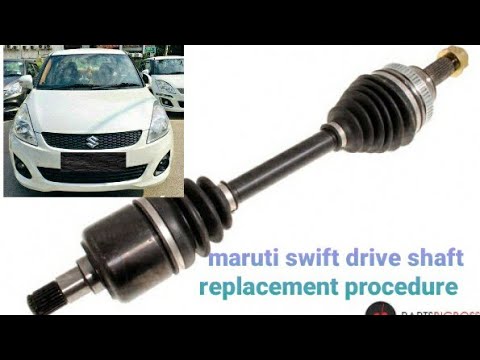This detailed infographic for car repair, featuring a Maruti Swift driveshaft replacement procedure, is encased between two black bars, one at the top and one at the bottom. The top left corner showcases a front-facing photograph of a white Maruti Swift, distinguishable by the 'S' on its grille, flanked by a white car on the right and a silver-gray vehicle on the left, all parked in a lot. Dominating the central portion of the image is an illustration of the driveshaft itself, displayed on a white background. This car part is a long, dark-colored metal rod with various components: rubber spirals, corrugated sections, and plain metal areas. Below the driveshaft, lavender and light aqua text clearly reads "Maruti Swift Driveshaft Replacement Procedure." Some text at the very bottom of the image appears cut off.